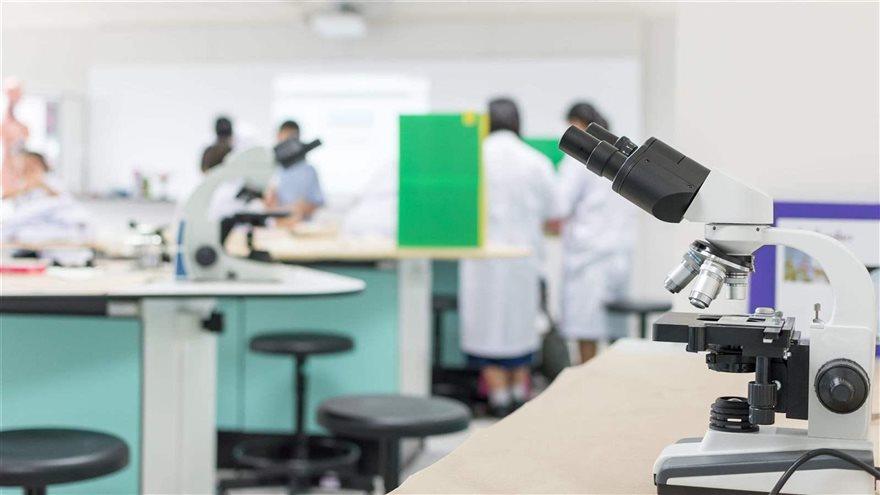The photograph captures a bright, bustling laboratory environment with several round tables and black stools scattered around. In the foreground, a white and black clinical microscope with binocular eyepieces, a turret housing multiple objective lenses, and bottom lighting sits unused on a table. The background, though blurred, reveals a lively scene with scientists in white lab coats gathered around various white workstations with teal bases, engrossed in their tasks. Among them, two additional microscopes, similar in model to the one in the foreground, can be spotted. The room features additional elements such as light fixtures, a photograph or possibly a poster on the wall, a mannequin, and a window in the background. There’s also an opening into another room where individuals not wearing lab coats are visible. A pinkish, indistinct object, perhaps an anatomical drawing, is partially visible to the far left.